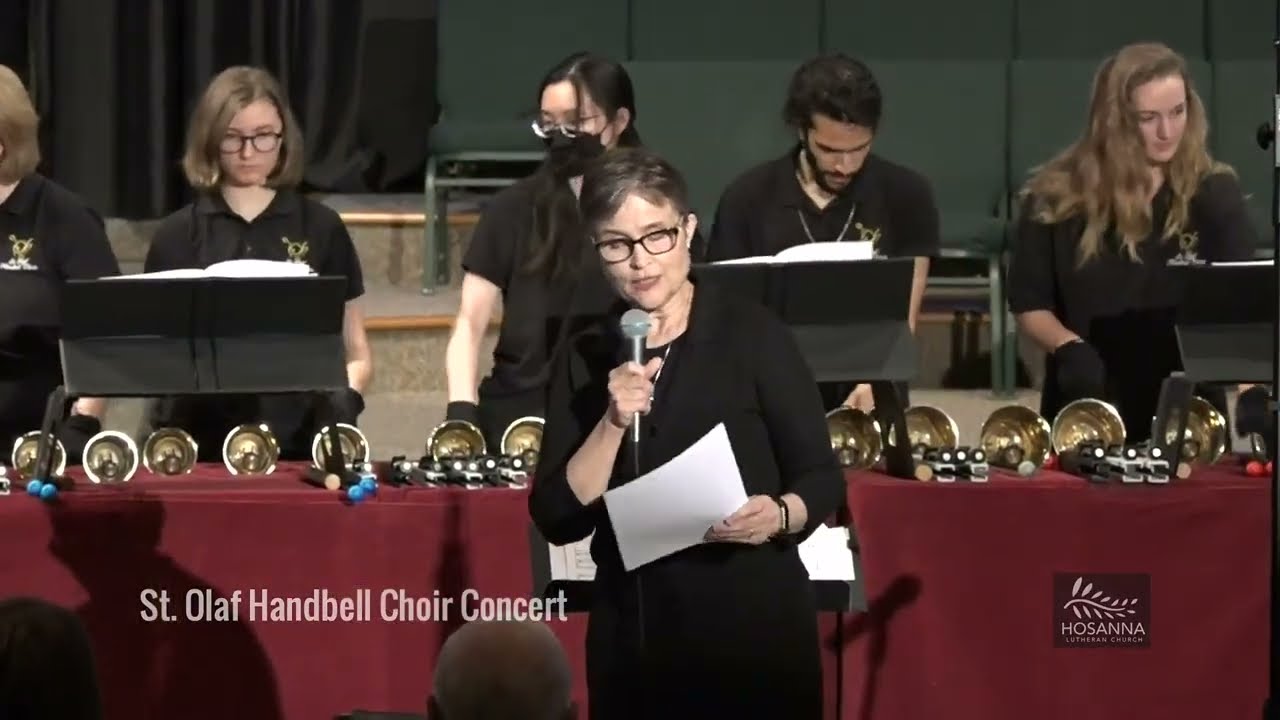In the image titled "Saint Olaf Handbell Choir Concert," a woman is seen standing on a stage, dressed in a black dress. She holds a piece of paper in one hand and a microphone in the other, speaking into it. She has short grayish-brown hair and black prescription glasses. Behind her, a long banquet-style table draped with a red tablecloth is adorned with assorted bells of various sizes. Seated behind this table are five individuals, all dressed in black short-sleeve polo shirts. Among them, four are females and one is a male. Two of the women and the man do not wear glasses, while two females sport eyewear. Notably, the female on the far right has long blonde hair, and one of the girls in the center is wearing a black PPE face mask. White text at the bottom left of the image identifies the event as the "Saint Olaf Handbell Choir Concert."